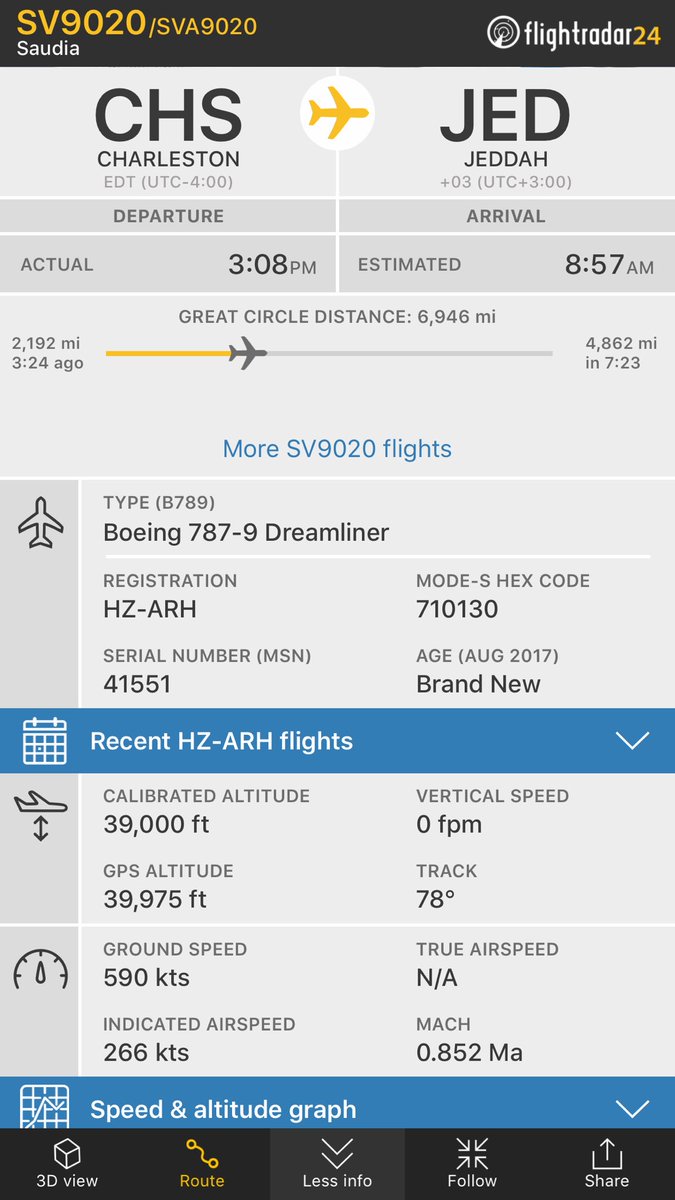Screenshot of Flight Radar 24 App Monitoring Saudia Airlines Flight SV9020

This detailed screenshot captures the interface of the Flight Radar 24 app on an iPhone. The top left corner identifies the flight as Saudia Airlines Flight SV9020. The plane departed from Charleston International Airport (CHS) under the Eastern Daylight Time Zone and is en route to King Abdulaziz International Airport (JED) in Jeddah. A small yellow plane icon represents the aircraft's position on the map.

The actual departure time was 3:08 PM, and the estimated arrival time across multiple time zones (UTC +03:00) is 8:57 AM. As of the screenshot, the flight has covered 2,192 miles over a duration of 3 hours and 24 minutes and has approximately 7 hours and 23 minutes remaining to reach its destination.

The aircraft is a modern Boeing 787-9 Dreamliner with the registration number H78-RH, manufactured in August 2017. Currently, the flight is cruising at a calibrated altitude of 39,000 feet. The app provides additional data such as ground speed, indicated airspeed, and true airspeed. Below this section—though not visible in the screenshot—a speed altitude graph is available for further insights.

At the bottom of the screen, navigation buttons include options for a 3D view of the flight, detailed route information, the ability to toggle additional information, a follow option, and share features.